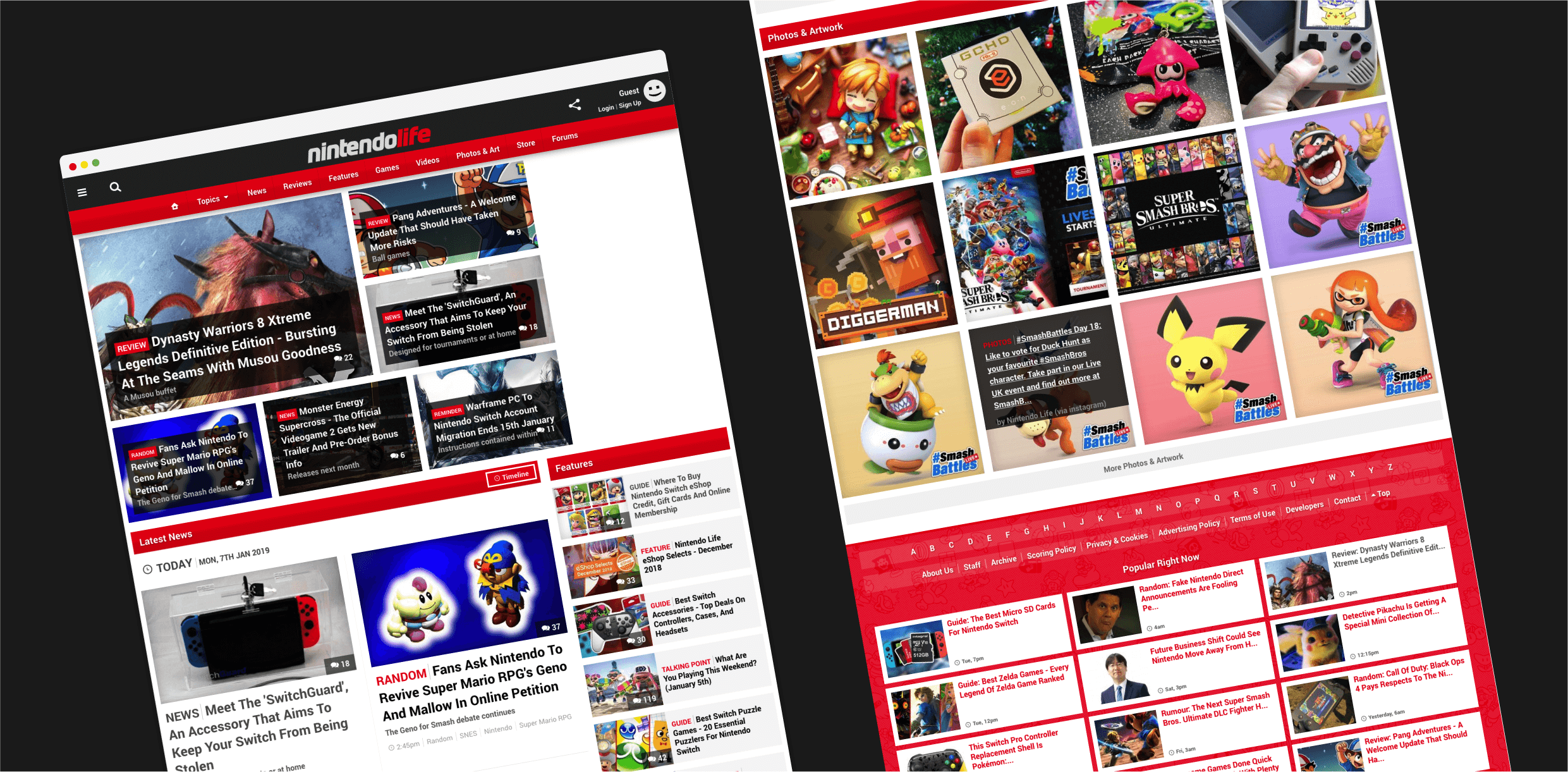The image features a digital interface set against a black background, displaying what appear to be two overlapping, partially cut-off web pages. The interface is shown on an Apple device, identifiable by the three colored circles (red, yellow, and green) in the upper left corner, indicative of the macOS window controls.

On the left page, the header includes three horizontal white lines, a white magnifying glass icon, and bold text that reads "Nintendo" in white followed by "Life" in red. It also displays user account options such as "Guest," accompanied by a smiley face icon, along with "Login" and "Sign Up" links in white text. A red navigation bar beneath this header lists several categories in white text: "Topics, News, Reviews, Features, Games, Videos, Photos, Art, Store, Forums."

Below the navigation bar are various game-related images and text blocks. One prominent text block in white reads, "Dynasty Warriors 8 Extreme Legends Definitive Edition. Bursting at the seams with M-U-S-O-U god goodness."

On the right page, various characters are depicted in dynamic poses. Notable among them is Pikachu, a yellow creature with black-tipped ears. Another character, likely the dinosaur figure from the Mario series, is shown above text that reads "Smash" in black and "Battles" in blue, followed by "Live." The bad guy from Mario is also visible among the characters.

This layered and dynamic image captures a vibrant, interactive interface filled with gaming content and character graphics.